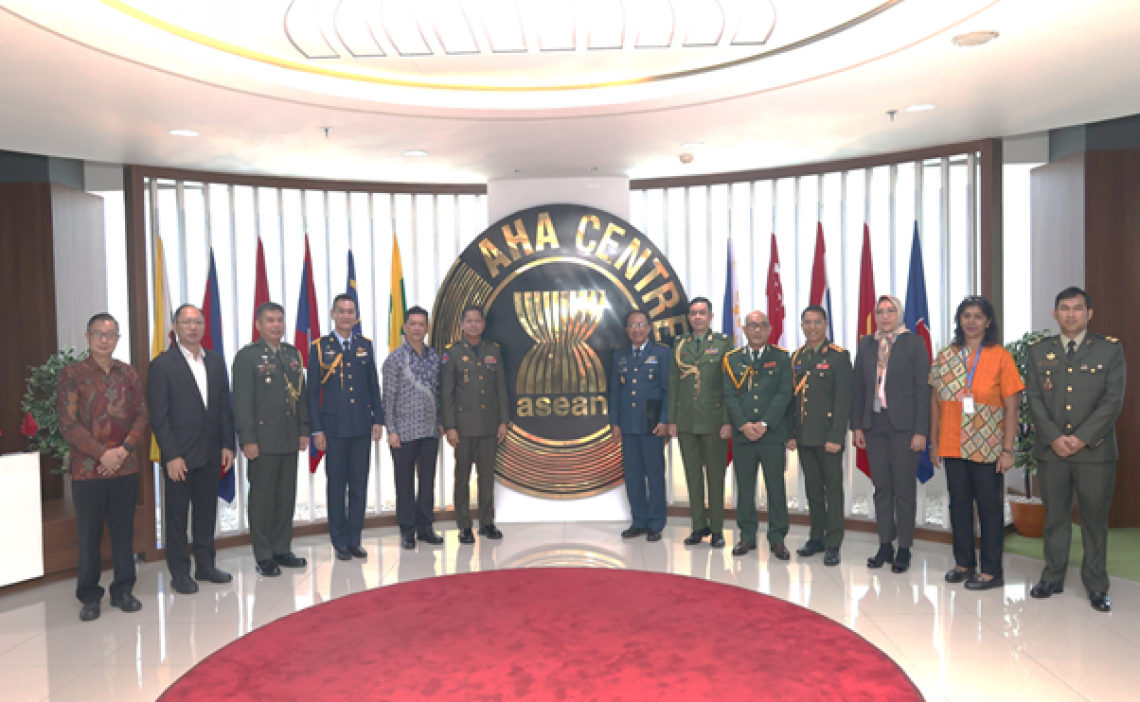This photograph captures a distinguished group of individuals standing around a wide circular window, posing in a semi-circle formation. The scene is set inside a government office, with a prominent emblem in the background that reads "AHA Center ASEAN" in gold letters against a black background, attached to a pillar. The group consists of six men in military uniforms on the left and seven individuals, a mix of military and civilian attire, on the right. They stand side by side in front of various national flags, symbolizing the diverse representation in the room. The polished white marble floor and the circular red rug in the foreground add an air of formality and elegance, complemented by the white ceiling above. The dignitaries' proud and distinguished demeanor underscores the significance of the moment captured in this photograph.